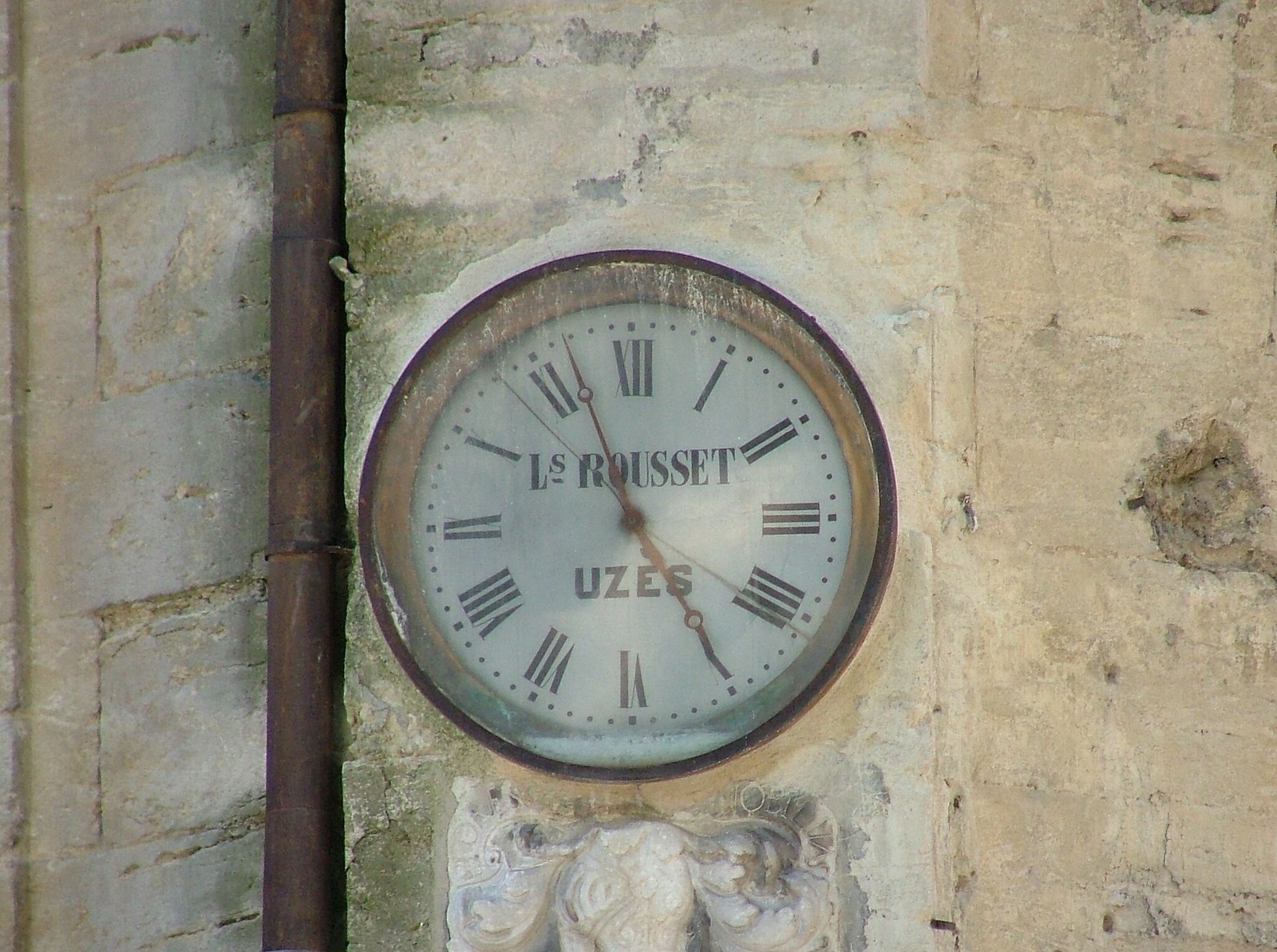This image captures an antique clock embedded into the side of a highly deteriorated stone building, possibly constructed from large, rectangular, tannish-white bricks. The ancient wall is marked with numerous cracks, stains, and broken pieces, adding to its weathered appearance. A slender, rusted cylindrical pipe runs vertically along the left side of the clock, contributing to the overall aged aesthetic.

The clock itself boasts a round face encased in a rusted metal border, suggesting it has endured many years of exposure to the elements. It sits in a white circle, protected by glass that shows signs of rain stains and wear. The clock face is adorned with black Roman numerals that indicate the hours, and the minute and hour hands are long, pointed, and made of reddish metal, with distinctive circular shapes about two-thirds down their length.

Prominently displayed on the clock face are the inscriptions "L.S. Rousset" and "Uzès," hinting at its origin in a non-English-speaking country. Just below the clock sits a weathered white sculpture, further enhancing the historic and artistic ambiance of the scene.